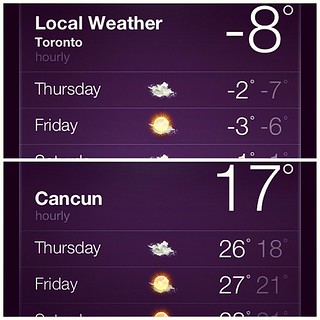A detailed caption for the provided image could read:

"A screenshot of the local weather application on a mobile device, displaying combined information from two instances of the app. The top of the screen is labeled 'Local Weather', with 'Toronto' prominently featured below. To the right, the current temperature in Toronto is indicated as -8°C. The forecast for Thursday and Friday is partially visible, with Saturday being slightly cut off. Both days are listed on the right side, accompanied by weather icons in the center, showing a cloud and the sun partially obscured by the cloud. For Thursday, the high is -2°C and the low is -7°C. For Friday, the high is -3°C and the low is -6°C. Below the Toronto forecast, a section provides the weather for Cancun, which is displayed as 17°C on the right side."